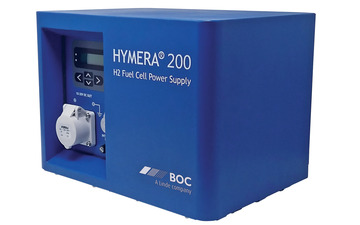The image depicts a blue, rectangular box product shot set against a stark white background. The box is labeled in white text on the top section: "Chimera 200 H2 Fuel Cell Power Supply." On the lower right-hand corner, the initials BOC, accompanied by a logo, indicate the manufacturer's name. A more detailed inspection shows an inset section on the left part of the box, featuring several buttons and a small digital screen. This section appears to be the interface for interacting with the power supply, including functionality such as turning the device on and connecting it to other equipment. This specific area includes illustrations, possibly white arrows, that guide users on how to operate the equipment.